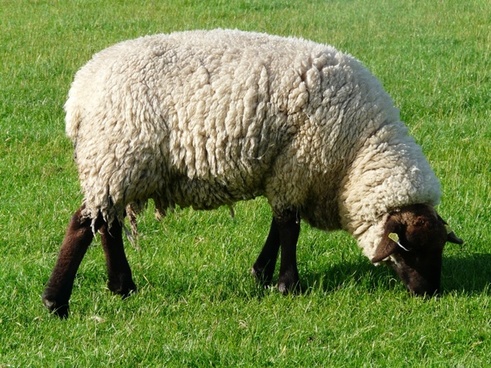In the photograph, a clean and remarkably woolly sheep stands contentedly in a lush, green field of grass. The thick, off-white wool coat of the sheep contrasts with its dark brown head and brown legs. Its head is lowered, grazing on the grass that is depicted as rich and thick, with a medium length and a vibrant green hue. The sheep’s pointed, triangular ears and dark hooves add to its characteristic appearance. The light source seems to be behind the sheep, casting its head in shadow and creating a darker area on the ground beneath its neck. Facing to the right side of the horizontal rectangular image, the sheep appears perfectly at ease, absorbed in its peaceful activity.